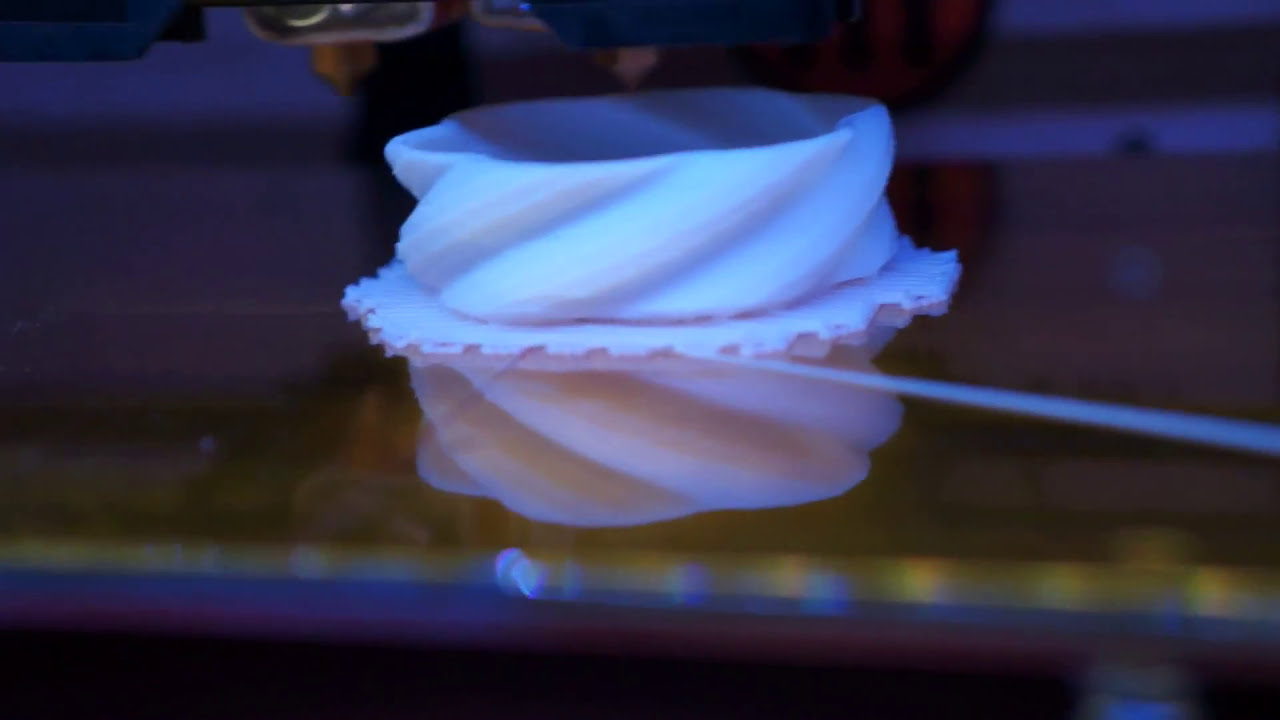This image captures a close-up view of a 3D printer in action, focusing primarily on the intricate creation being printed. The central object, a white, twisted spiral column, is positioned on a reflective surface that suggests a glossy, likely amber-hued tabletop. The twisted shape of the column displays delicate craftsmanship with subtle shades of pale blue and mauve-like streaks. Underneath this object appears to be a mat or doily-like material, possibly used to secure the object during printing. The lower portion of the frame transitions into darker tones with horizontal stripes of black, dark purple, and dark blue. The surface beneath the column exhibits a blend of dark yellow, purple, and maroon hues, adding depth to the scene. Above the object, you can discern the needle of the 3D printer, poised in its task of meticulously constructing the spiral shape layer by layer, illuminated by soft, subdued lighting that keeps the background minimally visible. Bright yellow and blue reflections add a touch of vibrancy to the edge of the reflective surface, completing this detailed snapshot of a work-in-progress 3D printed creation.